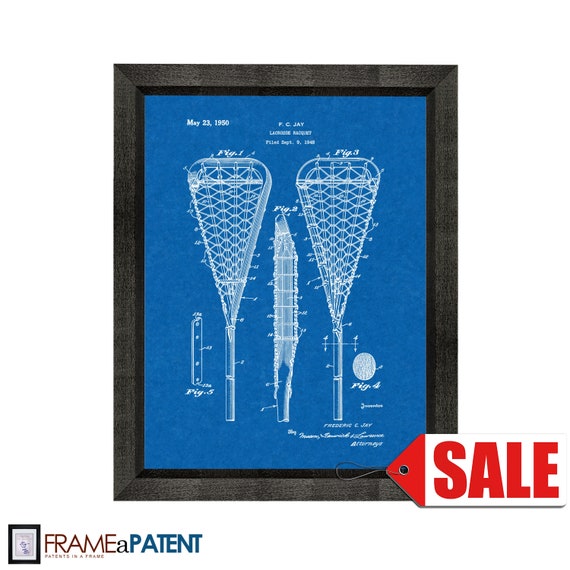A detailed and cohesive caption combining all given descriptions:

In this photograph, we see a patent drawing, dated May 23, 1950, enclosed in a simple wooden frame with a brown finish. The primary background color of the drawing is blue. The lower left corner features a smaller depiction of the frame labeled "FRAME" in large brown capital letters, accompanied by an "A" in small font, and adjacent to it, "PATENT" is written in large blue capital letters. The main design showcases two large, balloon-like structures flanking the sides, which resemble hot air balloons. These structures taper downwards, forming funnel-like shapes, and each has a notable feature: the right-hand structure includes a white circle near its stem. Between these main figures, there is a shorter, vertical, knife-like object also colored white. Additionally, a small vertical drawing on the left might represent a detailed section of the balloon-like design, and the text "Figure 5" appears beside it, while "Figure 4" is labeled on the round object on the right. Below these figures, there is descriptive text presumed to explain the patent details. A sail tag labeled “SALE” in red letters on a white background is attached to the bottom of the drawing, and the text "FRAME A PATENT" is displayed to the bottom left. The initials "FCJ" and the letters "P, C, and J" also appear on the image. The overall presentation gives the sense of a framed drawing of a patent, potentially depicting an aspect of either a lacrosse net or another netted item, although the exact item remains somewhat ambiguous.